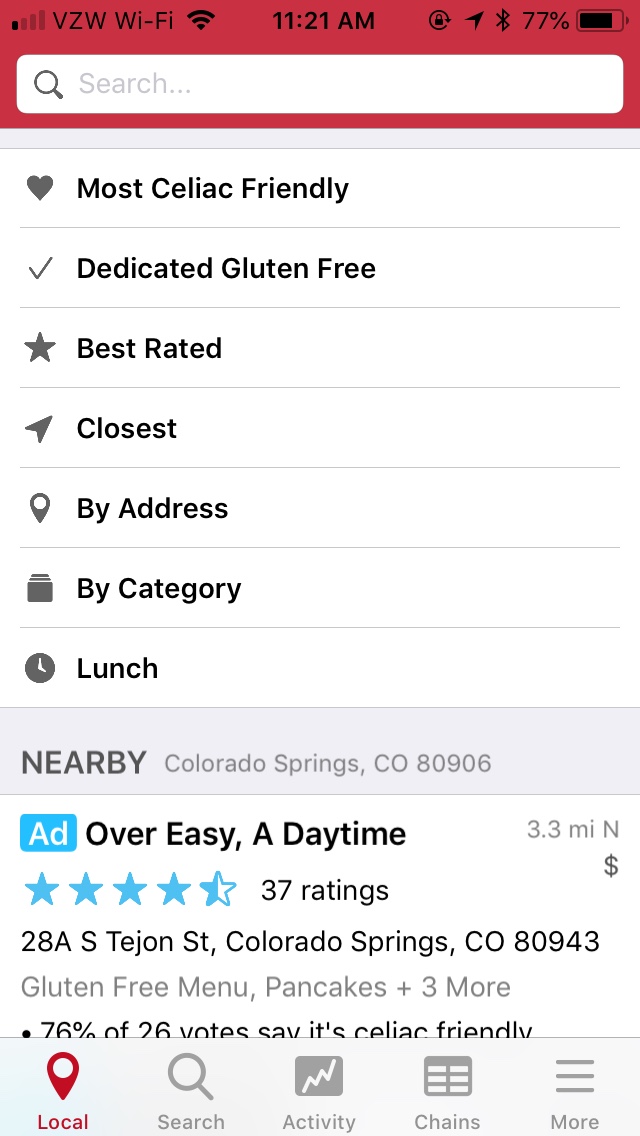This screenshot captured from a cell phone screen features an app interface with a prominently displayed red bar at the top, containing a blank white search bar. Below the search bar, the interface is organized into several informative sections, each accompanied by relevant icons:
 
1. A heart icon labeled "Most Celiac Friendly."
2. A check mark icon labeled "Dedicated Gluten-Free."
3. A star icon labeled "Best Rated."
4. An arrow icon labeled "Closest."
5. A pin icon labeled "By Address."
6. A shopping bag icon labeled "By Category."
7. A clock icon labeled "Lunch."

Additionally, below these sections, the location "Nearby Colorado Springs, Colorado 80906" is displayed, followed by an advertisement highlighted with a blue border. The advertisement promotes "Over Easy, A Daytime" restaurant, boasting a rating of four and a half stars from 37 reviews. The ad also mentions a gluten-free menu featuring pancakes and three more items, stating that 76% of 26 votes confirm it as celiac friendly.

At the bottom of the screen, there are navigation icons, with the "Local" tab being active, indicated by a red highlight and a pin icon.